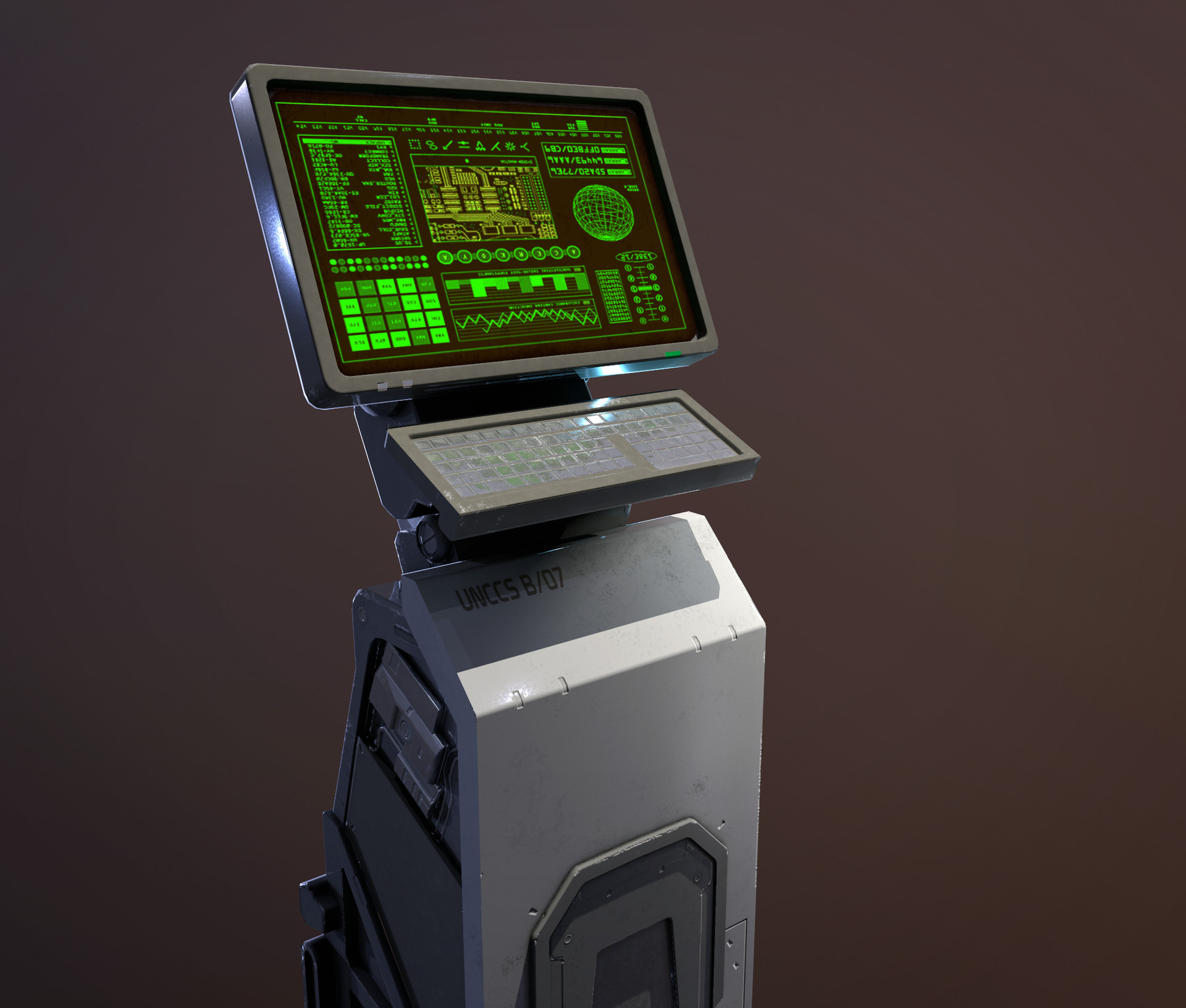This detailed color photograph captures a futuristic medical or scientific device against a dark brownish-tan, almost maroon background. The centerpiece is a sophisticated silver-gray machine featuring a rectangular monitor with a sleek silver border. The monitor itself displays an array of unreadable green text and charts against a black screen, giving the impression of high-tech data analysis or medical readouts. Prominently, there is a neon green sphere on the right side of the display, evocative of a globe. The screen is populated with various data visualizations including bar charts in the bottom middle and other charts and numbers scattered throughout, enhancing the complexity of the interface.

Below the monitor, there is a keyboard, though the specific letters are not discernible. The base of the machine is inscribed with "UNCCSB-07," suggesting a model number or designation. Additionally, there are various buttons and boxes on the left side of the display, indicating interactive components of the device. The overall aesthetic of the machine is highly advanced, reminiscent of equipment used for detailed medical diagnostics or intricate scientific research, invoking a strong sense of futuristic technology.